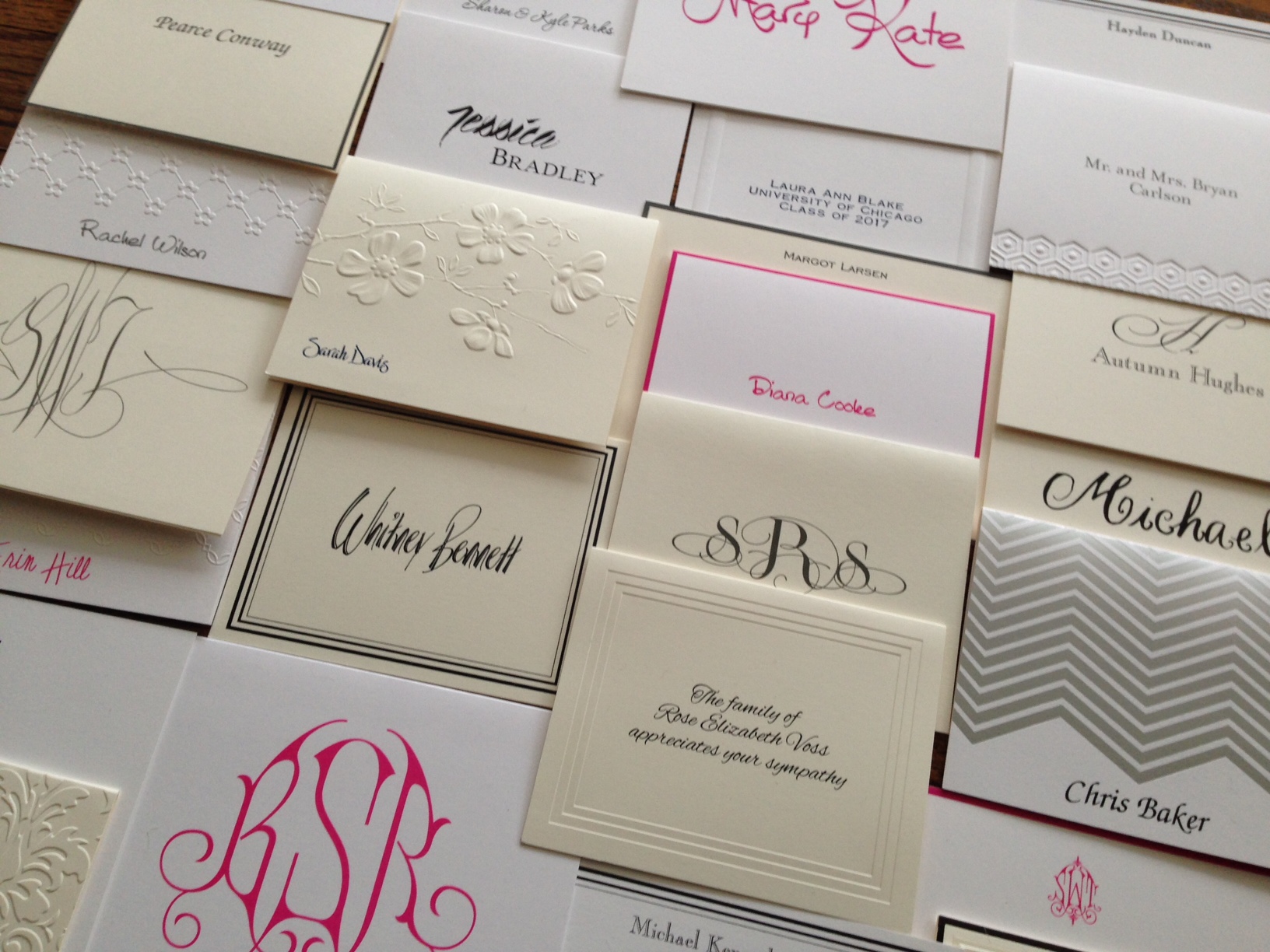The image is a horizontally rectangular display of note cards of various kinds in a shop, arranged neatly in columns and rows with multiple cards in each row. These cards can be personalized, featuring numerous designs, names, and initials. In the lower left corner, there's a card with red initials "RSR". Directly above it, another card has a black border and the name "Whitney Prescott." Further up the same column, there's a card with an embossed name at the bottom, followed by a white card bearing the name "Jessica". 

Other notable cards include a cream-colored card expressing sympathy from "the family of Rose Elizabeth Voss," and a card in the top row with the name "Pierce Conway". A variety of names can be seen across these cards, such as "Whitney Bennett", "Diana Cooley", "Mr. and Mrs. Brian Carlson", "Marie Kate", "Jessica Bradley", "Pierce Conway", "Chris Baker", and two cards with the name "Michael". Some cards are decorated with embossed flowers, initials like "BSR" and "SRS", and various other stylistic elements. The cards, mostly white or cream with black or pink writing, allow for a personalized choice in style and design.